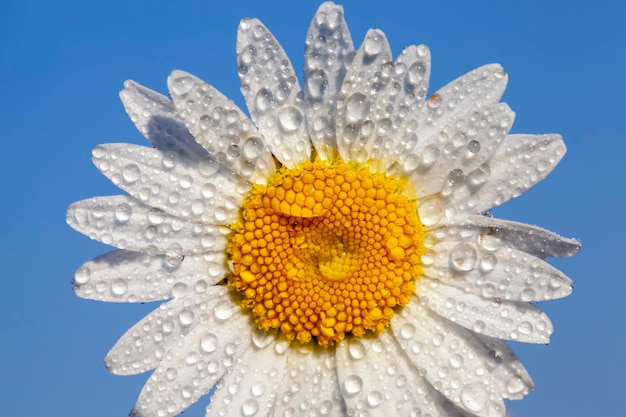This captivating photograph features a white daisy, covered in glistening droplets as if freshly sprayed with water. The daisy, centered in the image, showcases around 20 to 25 pristine white petals radiating outward from its core. The background is a clear, cloudless blue sky, enhancing the flower's pristine beauty. The flower's vivid yellow center, which contains tiny pollen spheres, is accented by small flecks of green. Notably, a large droplet of water rests prominently in the middle of the yellow center, magnifying the delicate pollen buds beneath it. Surrounding this focal droplet are numerous smaller droplets scattered across the white petals, creating a stunning, dewy appearance. The petals, arranged in layers, stretch slightly beyond the frame, giving the flower an expansive and lively presence.